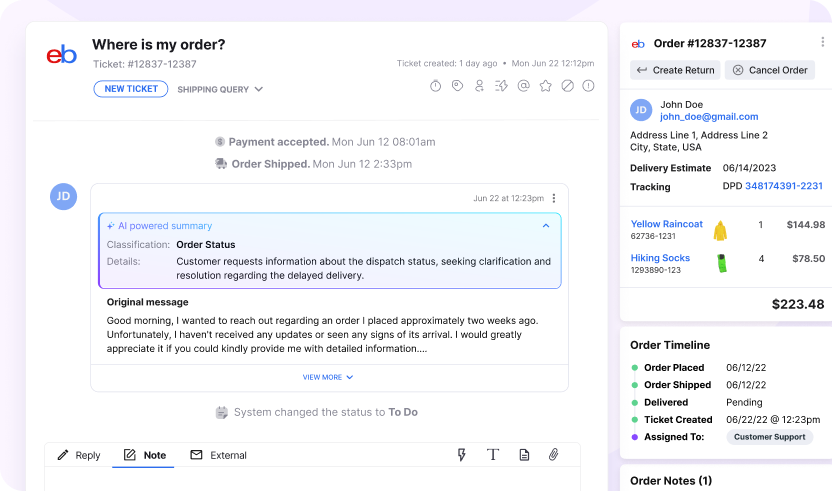**Screenshot of an eBay Order Inquiry Email**

In this image, there is a detailed screenshot of an email conversation related to an eBay order, set against a light purple, almost lilac, background. The screenshot features two windows.

**Larger Window (Left Side):**

- **Header:** At the top, in bold black text, it reads "Where is my order?" accompanied by the eBay logo, where the 'e' is red and the 'B' is blue.
- **Ticket Information:** Below the header, it lists the ticket number "12837/12387," the type of query "New Ticket: Shipping Query," and details regarding ticket creation, payment acceptance, and order shipment date.
- **AI-Powered Summary:** A smaller section with a user icon labeled "JD" describes the summary classification as "Order Status Details," highlighting a customer request for information about the dispatch status and seeking resolution regarding a delayed delivery.
- **Original Message:** The customer's message reads: "Good morning, I wanted to reach out regarding an order I placed approximately two weeks ago. Unfortunately, I haven't received any update or seen any signs of its arrival. I would greatly appreciate it if you could kindly provide me with detailed information."

**Smaller Window (Right Side):**

- **Action Options:** Includes buttons labeled "Create Return," "Cancel Order," and the customer's name and email: John Doe (john_doe@gmail.com).
- **Shipping and Contact Information:** Lists John's address, delivery estimate of "06/14/2023," and a tracking ID.
- **Ordered Items:** Includes order details with small images:
    - A yellow raincoat 
    - Hiking socks
- **Order Timeline:** Details the stages of the order - from placement, shipment, delivery status, to the creation and assignment of the ticket.

This vivid portrayal effectively communicates the sequence of events and the customer's concerns regarding the delayed order.